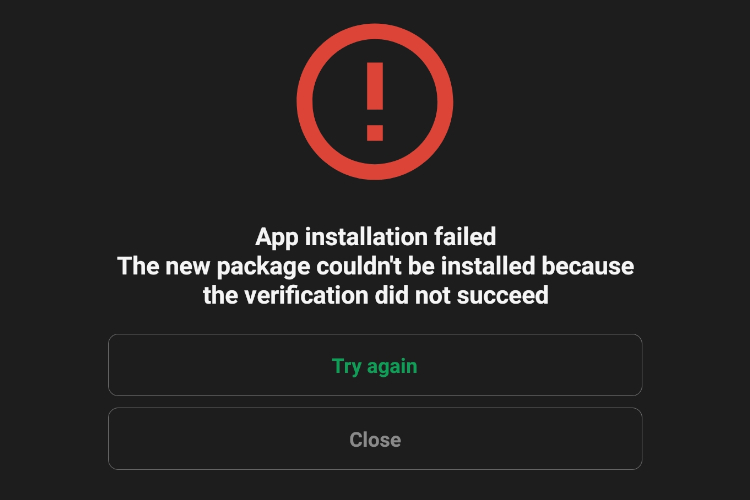The image depicts a large black notification box, centered prominently on a neutral background. The black rectangle lacks any decorative trim or borders. At the top, a vivid red circle encapsulates a bold, red exclamation point, serving as a striking warning symbol.

Beneath this symbol, the text "App installation failed" is displayed in white, with all elements center-aligned. Following that, another line of white text reads: "The new package could not be installed because the verification did not succeed" — notably missing a period at the end.

Further down, two centrally-aligned rectangles, providing functional options, are positioned. The upper rectangle, in bold font, reads "Try Again," with "Try" capitalized, indicating an option to attempt the installation process once more. The lower rectangle, colored gray to convey a sense of resignation, reads "Close," with "C" capitalized, offering the user an option to exit and abandon the installation attempt. Both options are padded with roughly an inch of space on each side, maintaining the centered layout and providing a clean, organized appearance.